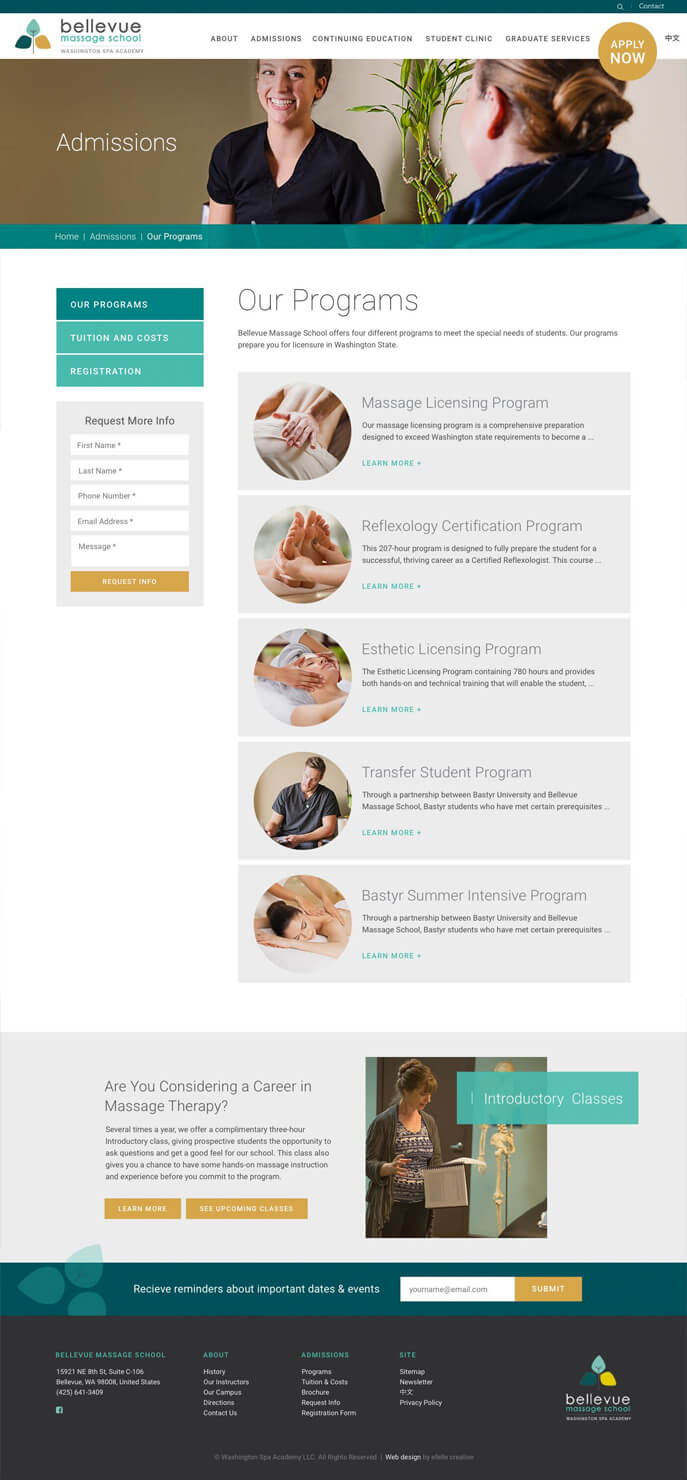Sure, here's a cleaned-up and detailed caption for the described image:

---

**Website Screenshot Overview:**

This image captures a full-page screenshot of a website, showcasing its entire layout from the top navigation bar to the bottom navigation bar. The predominant color theme is white for the background, complemented by various accent colors.

1. **Top Navigation Bar:** 
   - There is a thin, dark green or dark gray line running across the top width of the site.
   - Below this line, a white navigation bar features the word "Bellevue" along with a company logo.
   - Tiny, unreadable font text likely lists the navigation options from left to right.

2. **Header Section:**
   - A prominent photograph serves as part of the header, capturing a smiling woman facing the camera and another woman with her back to the camera.
   - The word "Admissions" is overlaid on a brown background next to the photograph.
   - A teal line beneath this section contains text that is not legible in the screenshot.

3. **Main Content:**
   - A smaller navigation bar is located on the left side.
   - On the right, the section is labeled "Our Programs."
   - Five gray blocks are lined up, each containing a circle with an image inside. These images likely pertain to categories such as massage, health, beauty, or spa services.

4. **Bottom Section:**
   - The bottom part features a gray block with some text and a photograph on the right.
   - A teal bar is situated below this gray block, containing a search bar and additional information.
   - At the very bottom, a dark gray section repeats the Bellevue logo in the bottom right corner, accompanied by traditional navigation links such as "Contact Us."

This comprehensive screenshot effectively displays the structure and visual elements of the "Bellevue" website, offering insights into its design and organization.

---

Feel free to adjust any specific details as needed!